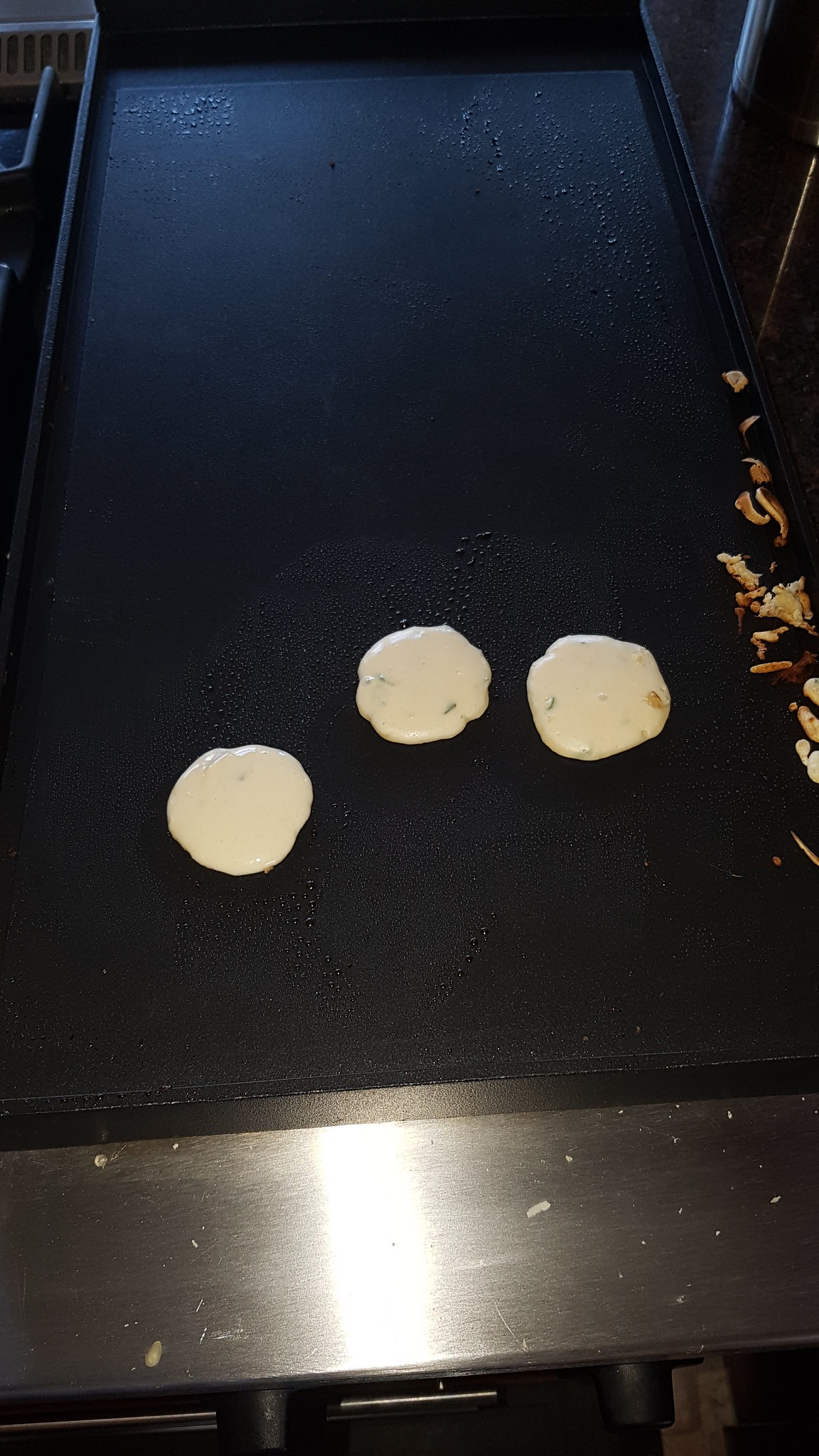This photograph captures a bustling moment in a commercial kitchen, focusing on a substantial, black cast iron griddle that likely spans about six feet in length and four feet in width. The griddle, sitting on a stainless steel range top with chrome detailing and black dials, dominates the scene. Reflecting light from above, the griddle's surface reveals its activity: three small, uncooked pancakes with bubbling batter, indicating the heat beneath them. To the right of these pancakes are remnants of previously cooked food, possibly hash browns or burnt pancake edges, adding to the sense of ongoing culinary action. The composition, while not perfectly framed, vividly conveys the dynamic environment of a professional kitchen.